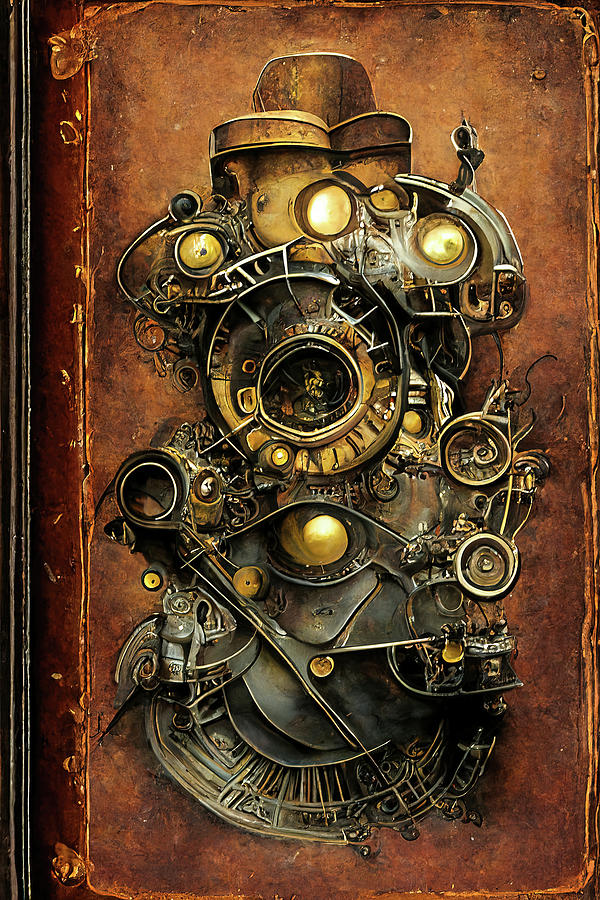The image is a highly detailed digital illustration resembling a cyberpunk-inspired sculpture of intricate mechanical parts. The sculpture, reminiscent of a fanciful machine or a multi-layered gear structure, features a complex arrangement of metal plates and disks intertwined and connected. Predominantly dark grey in color, it also includes elements of gold chrome, lending a striking contrast. The assembly forms a shape akin to a fire hydrant or possibly a figure, with a rounded globe suggestive of a head and an off-kilter eye formed from various machinery elements. At the top, what appears to be a brimmed hat made of metal crowns the structure.

The background is a rich, textured mix of dark brown with dark red borders, evoking the appearance of an ornate, worn-out book cover. This lends the entire piece a regal, almost antique feel, as if it could be the cover of a royal tome. The sculpture is punctuated by a large black circle at the base and smaller metallic components, including little silver tubes and circular gold accents. It convincingly blends three-dimensional aspects, giving it a substantial, tangible presence despite its digital nature.